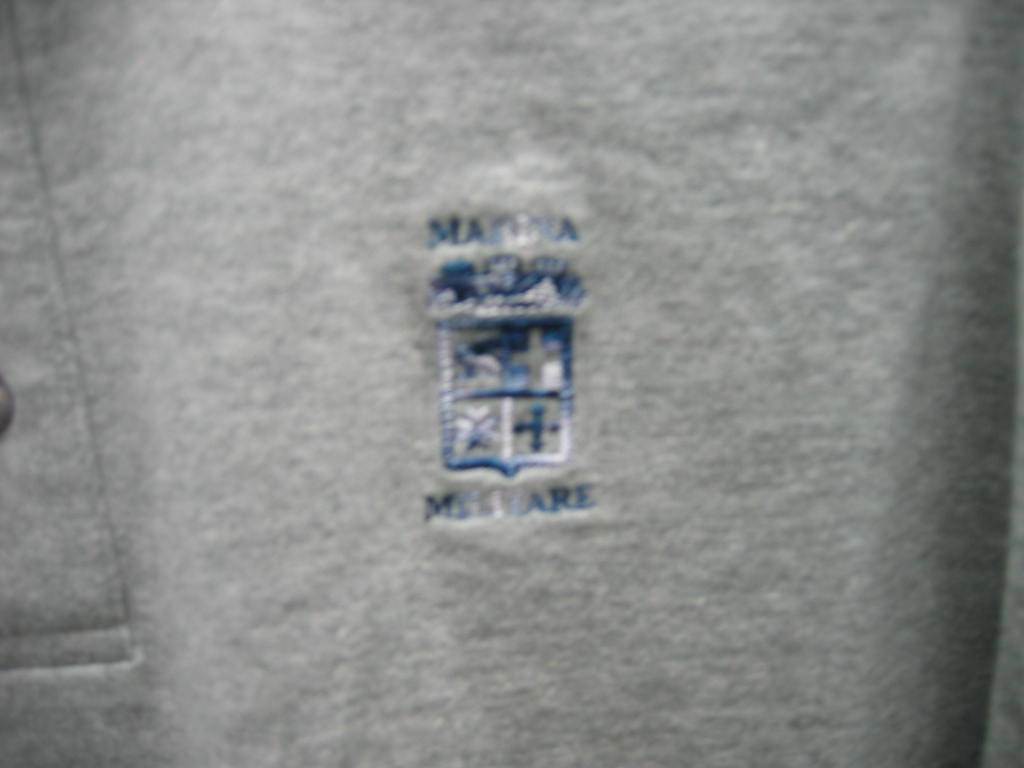This is an up-close photograph of a logo embroidered on a gray Henley shirt. The detailed embroidery, in fine blue and silver threads, forms a rectangular crest or shield. The top and bottom of the logo feature words that begin with the letter 'M'. The upper half of the emblem includes a silver cross on a blue background, flanked by what might be a ribbon or an eagle. The crest contains three compartments: the bottom right quadrant distinctly displays a blue cross. Surrounding the emblem are careful stitch lines, with one vertical stitch running from the upper left corner and a horizontal stitch that meets it near the bottom left edge of the image. On the left edge of the photo, the edge of a brown button is visible, suggesting this could be a Henley shirt. The precise details and colors of the logo, despite some blurriness in parts, hint at a possible military affiliation.